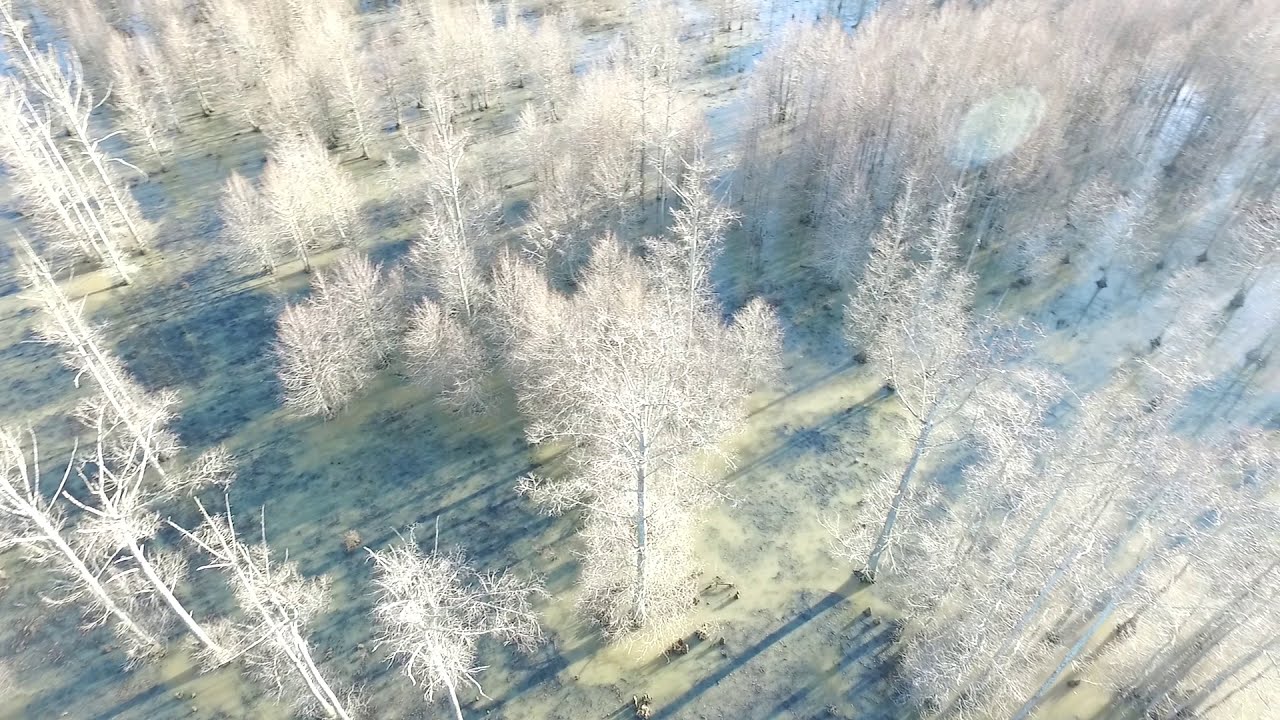This is an aerial view of a seemingly eerie deciduous forest blanketed in snow or covered in frost. The trees, standing straight with their limbs and branches appearing stark white, cast shadows that fall to their left, suggesting the sun is shining brightly from the right, even though the sky itself is not visible. The forest floor shows an unusual mix of colors—patches of yellow, very light green, and hints of blue—possibly indicating a flooded area with water mixed with mud, adding to the surreal and almost negative-like appearance of the landscape. Scattered across the scene are occasional black spots at the base of some trees, likely where the trunks meet the ground. The shadows stretch horizontally or diagonally, enhancing the feeling of an enchanting, wintry forest.